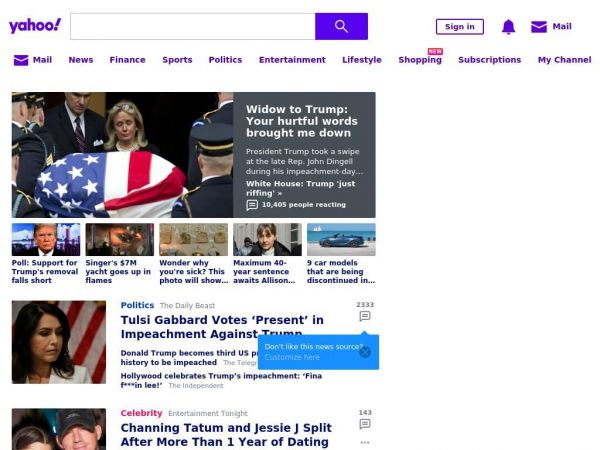This image, sourced from a Yahoo search, prominently displays the Yahoo logo in purple at the top of the page. The top navigation bar features links to various sections: Mail, News, Finance, Sports, Politics, Entertainment, Lifestyle, Shopping, Subscription, and My Channel.

The central focus of the image is a poignant news story headline that reads, "Widow to Trump: Your hurtful words brought me down." In the image, a grief-stricken woman stands in front of a casket draped with the American flag, clearly in mourning. Her tear-streaked face and sorrowful demeanor underscore her deep sadness. Surrounding her are servicemen respectfully carrying the casket. 

The associated news blurb mentions that President Trump made derogatory remarks about the late Representative John Dingell during his impeachment proceedings. Below this primary story, there is a set of five small thumbnail images with captions beneath them, accompanied by two larger images on the right side of the screen.

At the bottom of the page, a blue box labeled "Don’t like this news source?" is displayed, with an option to customize content by clicking a designated area.